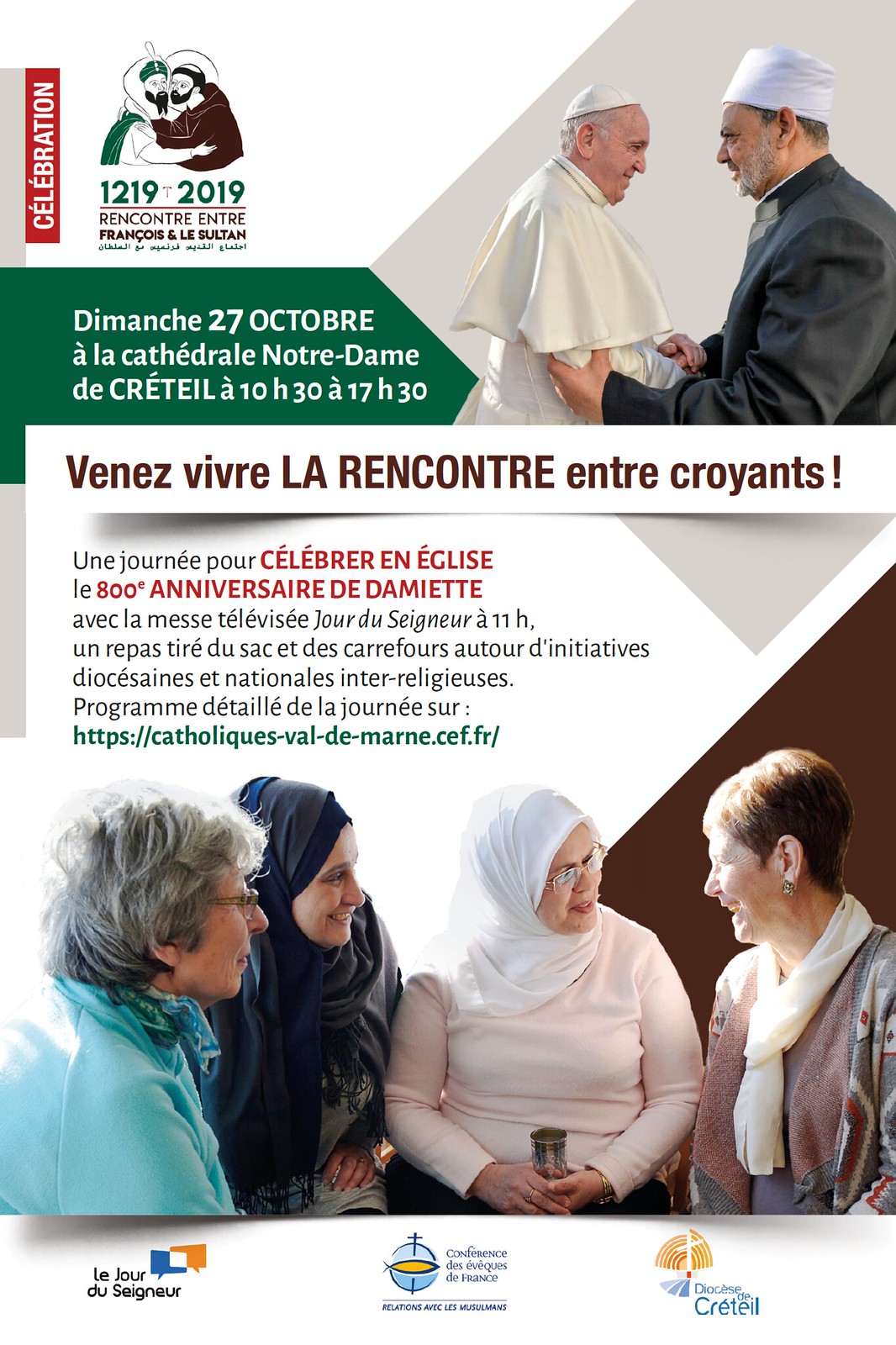This image appears to be a digitally-rendered infographic promoting an event commemorating the 800-year anniversary of a historic meeting. The top section features a notable image of Pope Francis in his white robes shaking hands and slightly embracing a Muslim religious leader, who is dressed in a dark gray jacket and a slightly looser white cap. Both figures are positioned against a gray background highlighted with geometric shapes and a green arrow pointing towards them. Above them, a vertical red banner with white text reads "Celebration," flanked by a logo of two people embracing and text that notes "1219 to 2019, Rencontre, Entre Francois et le Sultan," suggesting a celebration of the encounter between Francis and the Sultan. Further event details, entirely in French, are displayed on the left side, mentioning "Dimanche, 27 Octobre, à la cathédrale Notre-Dame," indicating the date and location.

The bottom section of the image showcases a photograph of four women in lively conversation. Among them, two are notably wearing headscarves, indicative of Muslim attire. One woman wears a white hijab paired with a white top and black pants, while another sports a blue hijab. The remaining two women, one with red hair wrapped in a white scarf and another with silver hair in a blue shirt, appear to be engaging attentively in the discussion. Several logos featuring crosses are located at the bottom, reinforcing the religious context of the event, which appears to be an intercultural and interfaith celebration at the Cathedral of Notre-Dame on October 27th.